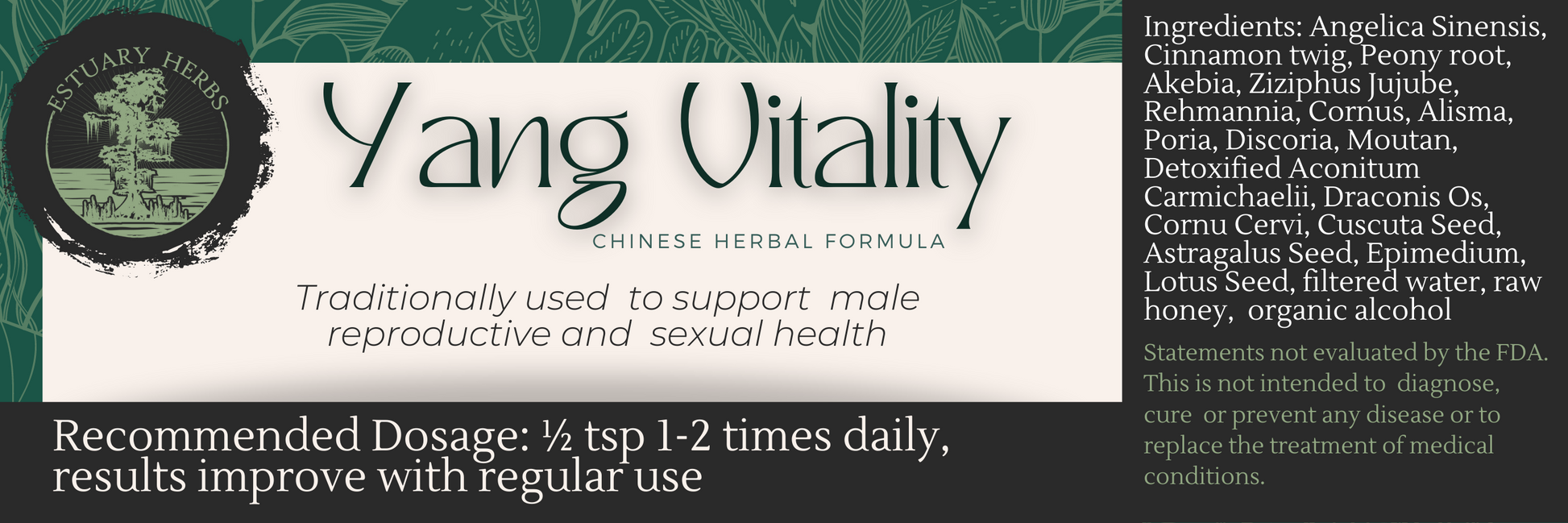The image depicts a label from Estuary Herbs for their product, Yang Vitality, a Chinese herbal formula traditionally used to support male reproductive and sexual health. The label's background is green, adorned with lighter green leaves. At the top left, the Estuary Herbs emblem features black text with light green words and a tree motif. The product name, "Yang Vitality," is written in black on a white banner, which is bordered by green with various leaves and greenery. Below the product name, a black strip displays the recommended dosage: "one-half teaspoon, one to two times daily," followed by the note that results improve with regular use.

To the right of the main text, the ingredients are listed in red on a black background: Angelica sinensis, cinnamon twig, peony root, akibia, zizifis, jujube, romania, cornus, elisma, poria, dysgoria, mountain, detoxified acanitum karmichaeli, draconis ose, cornucervae, cacusta seed, astragalus seed, epitomeum, lotus seed, filtered water, raw honey, and organic alcohol. Below the ingredient list, a disclaimer is printed in green on the black background: "These statements have not been evaluated by the FDA. This product is not intended to diagnose, cure, or prevent any disease, or to replace the treatment of medical conditions."